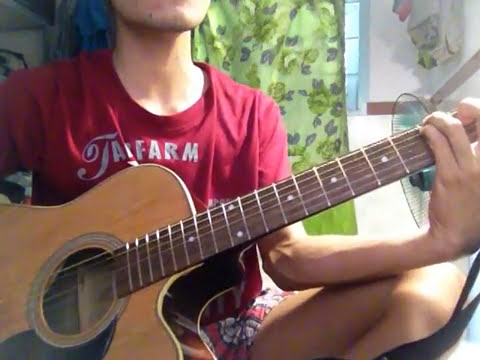The photograph captures a young, slender person playing an acoustic guitar, positioned predominantly on the left side of the image. Their face is not visible, as it is cropped out from the chin upwards, allowing only a view from their chin to part of their legs. They are seated and clad in a red short-sleeve t-shirt adorned with white handwritten text that appears to read "Tap Farm" or "Jai Farm." Complementing their shirt, they are wearing red, black, and white Hawaiian-style shorts. The guitar they are holding is a tan, wood-grain acoustic with a darker brown or black pick guard. The person's right hand is poised on the neck of the guitar, suggesting they are playing a chord.

In the background, a green floral curtain decorated with a pattern of flowers and leaves partially covers a window, letting in some light and revealing a glimpse of green trees outside. The backdrop also includes a white wall adorned with what appears to be a white poster or picture, and in the top left corner, something blue is hanging. Additionally, there’s an oscillating fan visible behind the person's left hand, adding to the detailed ambiance of the room, which could likely be a bedroom.